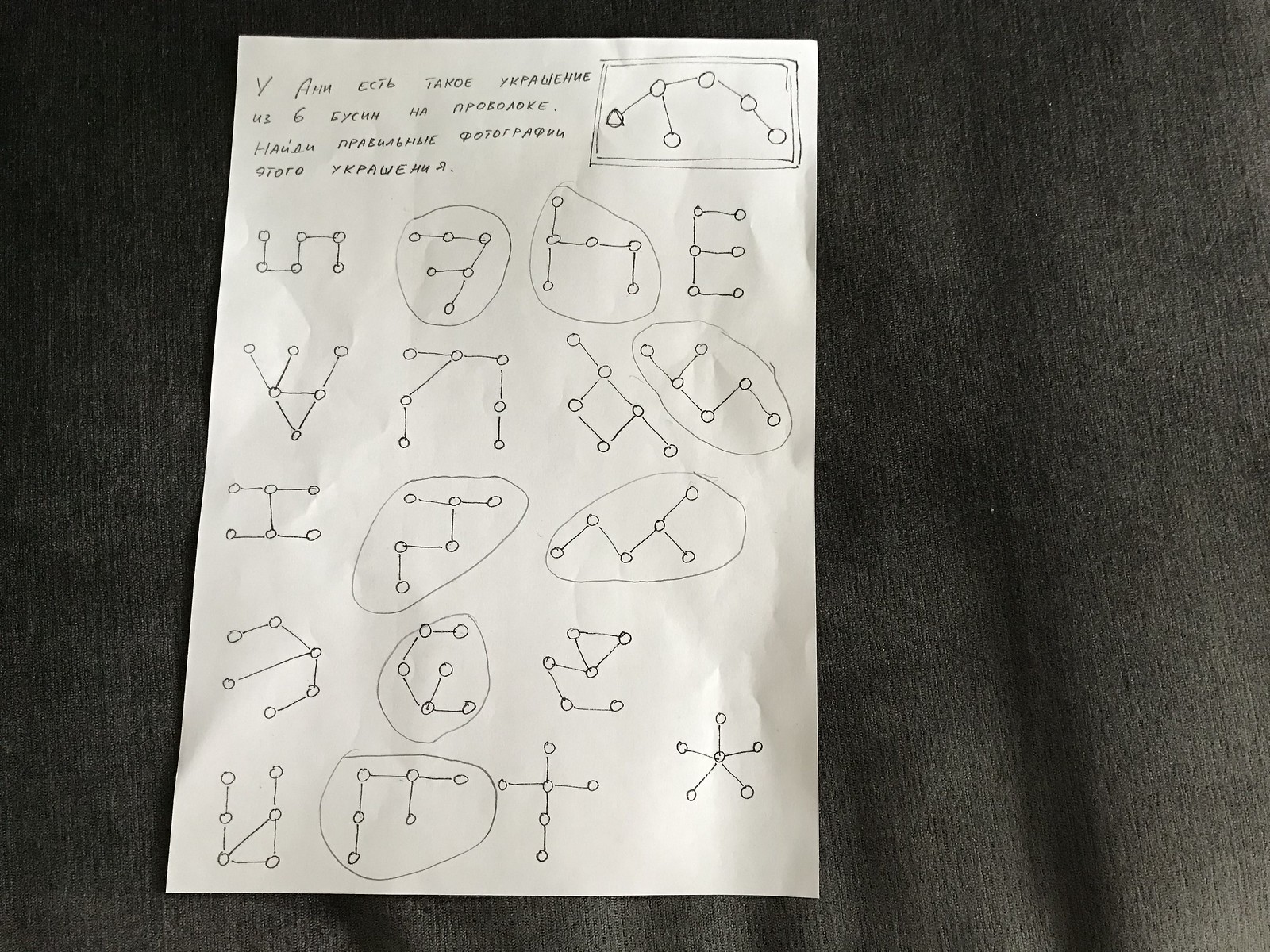In this image, we see a drawing on a piece of white paper, approximately nine inches in height. In the upper left corner, written in pen, the text begins with what appears to be a "V" followed by an uppercase "A." The rest is somewhat blurred and difficult to read. Further along, the word "TANOE" becomes discernible, followed by more indistinct letters. On the second line, the word "us" is clearly written, followed by the number "6" and a series of letters that do not form any recognizable word. The bottom row also contains a sequence of letters that do not seem to spell out any specific word.

To the right of this text is a detailed drawing enclosed within a rectangle. The drawing consists of five dots on the top row, all connected by lines. A line descends from the second dot on the top row and connects to another dot, forming a web-like structure. There are four rows of these interconnected dots and lines, with lines extending in various directions. Notably, circled dots appear at several points within this structure: two on the top row, one on the second row, two on the third row, one on the penultimate row, and the second dot on the very last row is also circled.